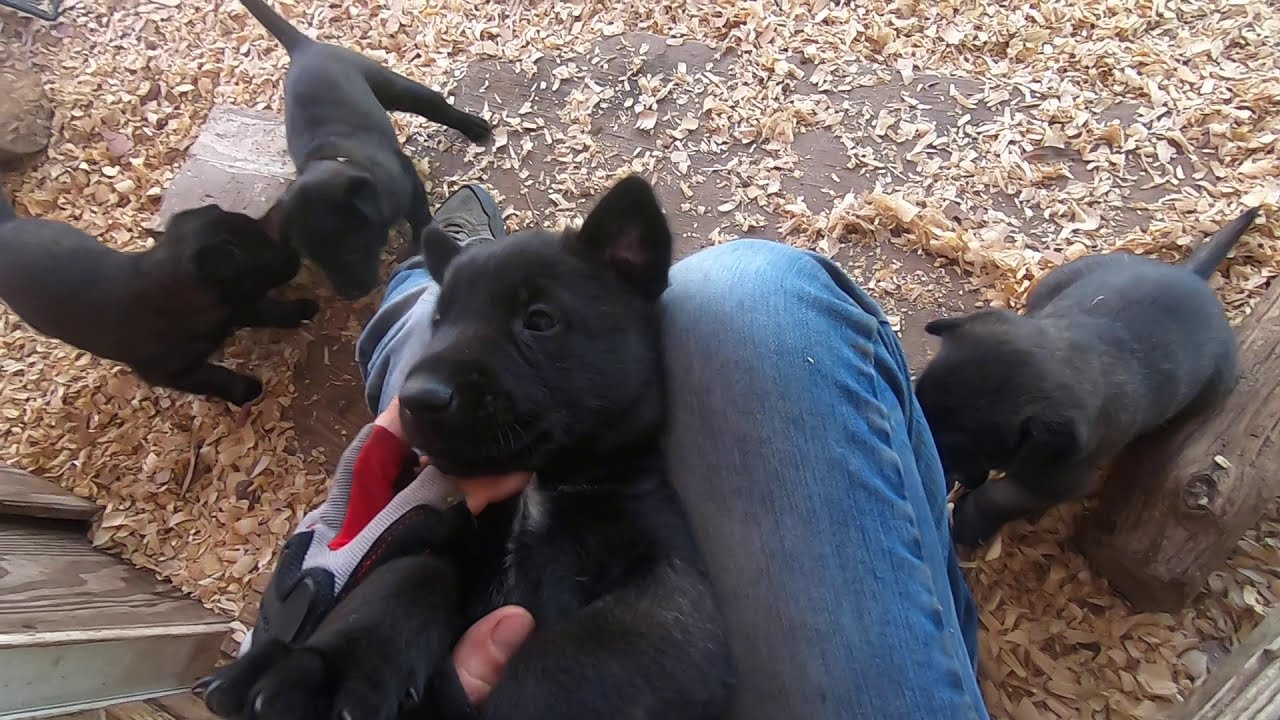In the partial indoor scene, a person dressed in blue jeans is holding a small black puppy with a little white on its neck atop their knees. The puppy, which has dark eyes and a dark nose, is lying on its back between the person's legs as they're petting it. Scattered around are wood shavings, creating a soft, textured floor. Beneath the person’s feet, another black puppy is partially visible, with just the top of its head, ears, and tail showing. To the left, two additional black puppies play together in the wood shavings. Various elements like a bowl, a brick, or pieces of cardboard can be seen amidst the sawdust, hinting that the setting might be a pen or an enclosed space.